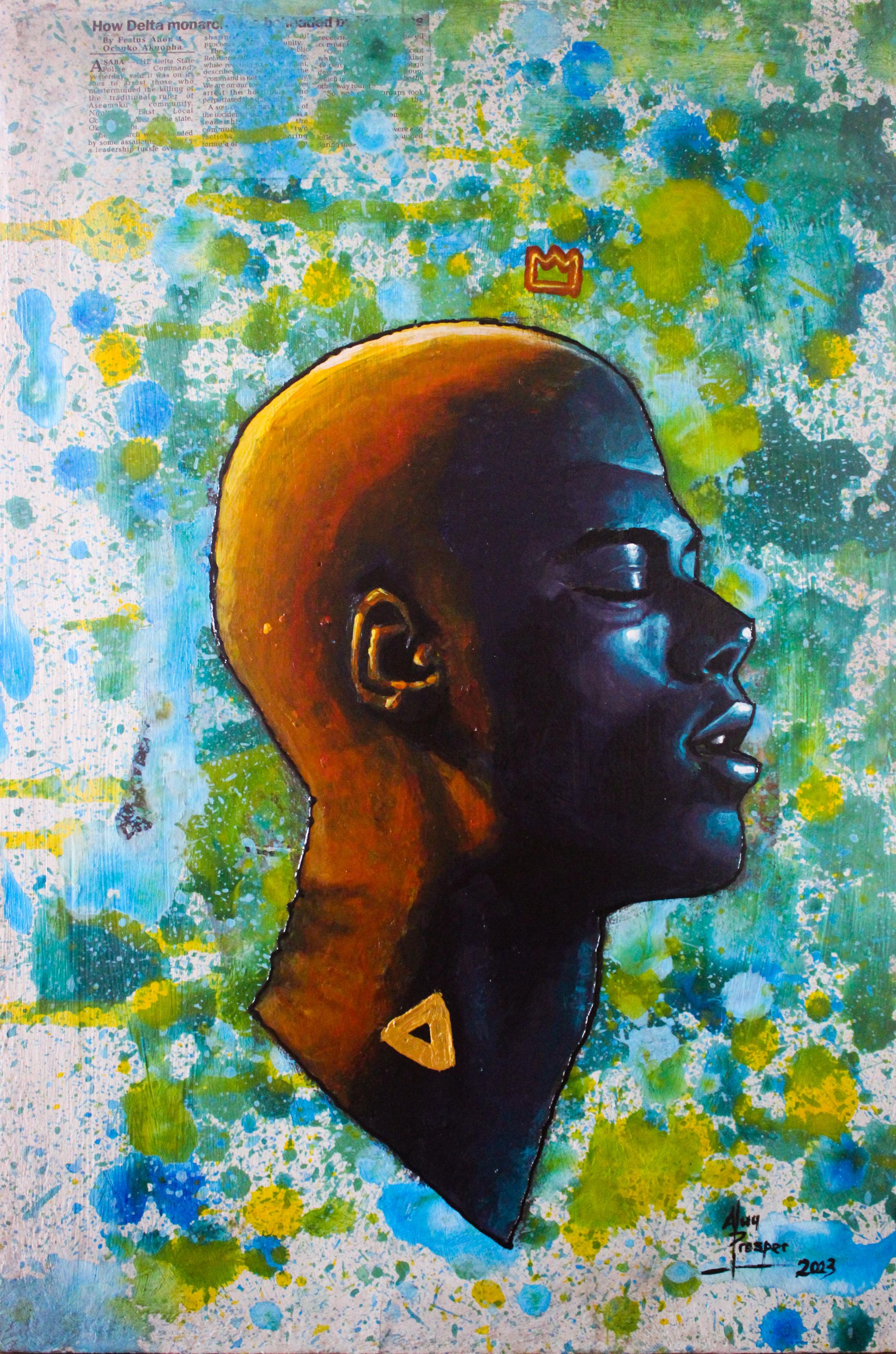This painting features the side profile of a bald African American man, depicted with a rich brown complexion transitioning to orange and yellow on the top of his head. His eyes are closed, and his slightly open mouth combined with an upward-turned nose suggest that he is lost in thought. The artist has added a small, golden crown hovering just above his head, not touching it. On his neck, a yellow triangle stands out, adding a geometric touch to the artwork. The background consists of a white canvas adorned with spontaneous splotches and dots of green, blue, and yellow, creating a vibrant, almost abstract environment. The man's face is accented with a subtle blue glow, enhancing the depth and shading. The piece is signed by the artist in the bottom right corner.